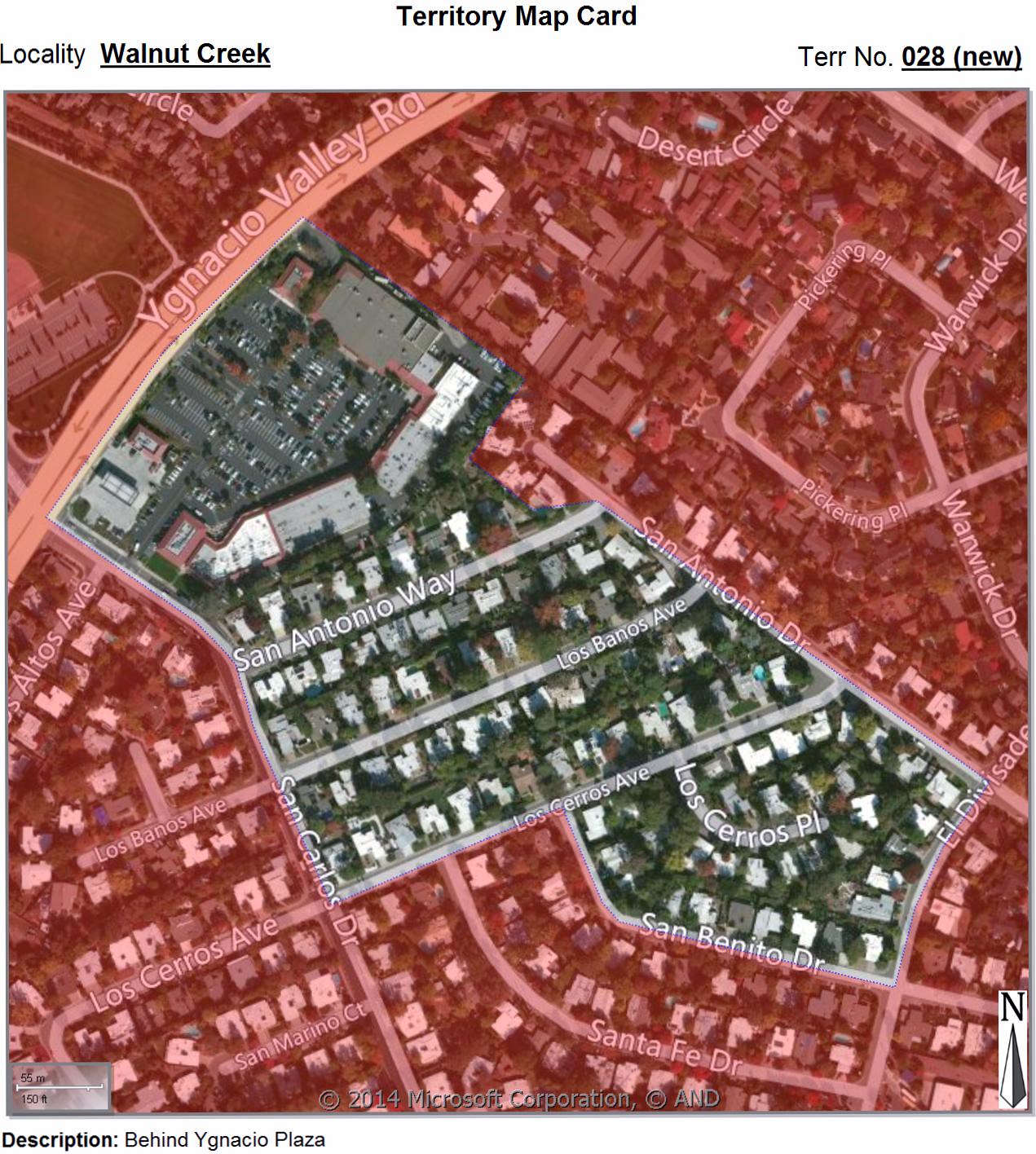The image depicts a screen capture of a map display, viewed from an overhead perspective. The central region of the map is highlighted in color, while the surrounding areas and roadways are marked in pink, clearly indicating that the central region is the primary focus. Several streets are labeled within this highlighted area, including San Antonio Way, Los Buenos Avenue, Los Creso Avenue, San Bernardino Drive, and Santa Fe Drive. These street names suggest a locale that could likely be in or near California.

At the upper part of the image, the word "locality" is featured, underlined by the name "Walnut Creek." In the center of the map, there is a label reading "territory map card," and to the right, it reads "TERR No. 028 (new)." Below this label, a description reads "Beyond YGNACIO Plaza." In the lower right corner of the image, there is an overlay featuring a compass indicator pointing north.

Additionally, to the upper left of the map, there appears to be a plaza area, which is suggested to be YGNACIO Plaza, a place likely to house various stores. This plaza is situated near YGNACIO Valley Road, a highway that further supports the identification of the area.